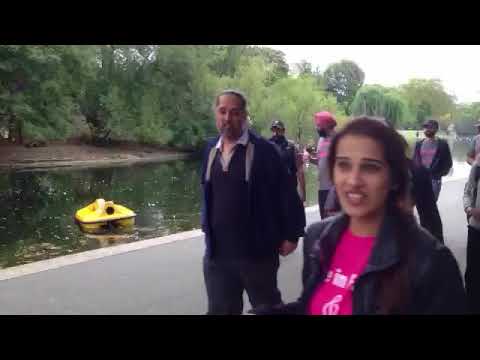In this outdoor photographic scene, a group of people walk along an asphalt path beside a serene canal. Dominating the bottom right corner is a woman, likely in her early 30s, who appears to be Hispanic or South Asian. Her dark hair gracefully falls over her shoulder, contrasting with her black blazer worn over a vibrant hot pink t-shirt. The partial lettering "IM" and a music symbol are visible on the shirt. To her left, an older South Asian man, perhaps in his 50s or 60s with a beard and mustache, walks alongside her. He wears a black jacket over a gray or blue shirt and dark pants. In the center background is another man of South Asian descent, distinguished by his red turban and beard, engaging in conversation with a man wearing a baseball cap. The canal to their right features a bright yellow boat floating quietly. The scene is framed by reflections of trees on the water and a grey, cloud-filled sky overhead, capturing a tranquil moment shared among diverse individuals.